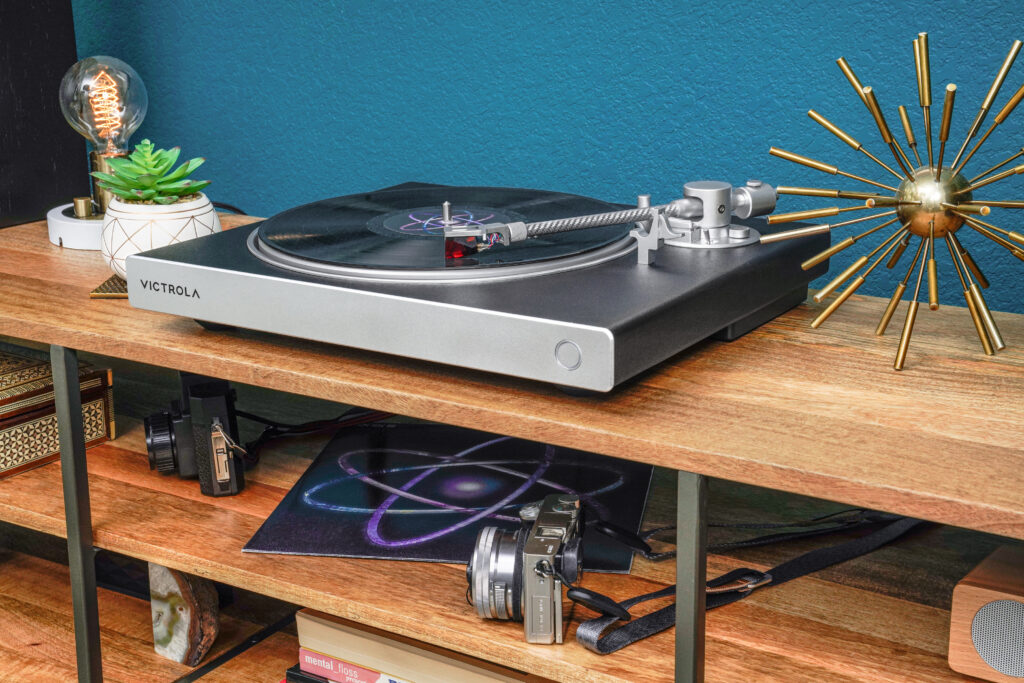This image depicts a wooden shelving unit against a blue wall, with three distinct shelves. On the top shelf, there is a modern silver Victorola record player, with a vinyl record loaded and a handle featuring a red needle. To the right of the record player, there is a golden sunburst decoration with metallic rays protruding outward. On the left side of this shelf, a small succulent plant is positioned next to a display encasing a vintage-style lightbulb. The upper right-hand corner of the image shows a gray area, the nature of which is unclear.

On the second shelf below, there are two cameras; one is an old black camera, and the other is a silver camera possibly from the 1980s. This shelf also holds a small square poster depicting an atom, two wooden boxes—one resembling a speaker and the other possibly a jewelry box.

The bottom shelf contains a series of horizontally stacked books and a rectangular marble prism. The shelving unit is constructed with brown wood and supported by black metal poles and legs, adding to its sturdy yet stylish appearance.